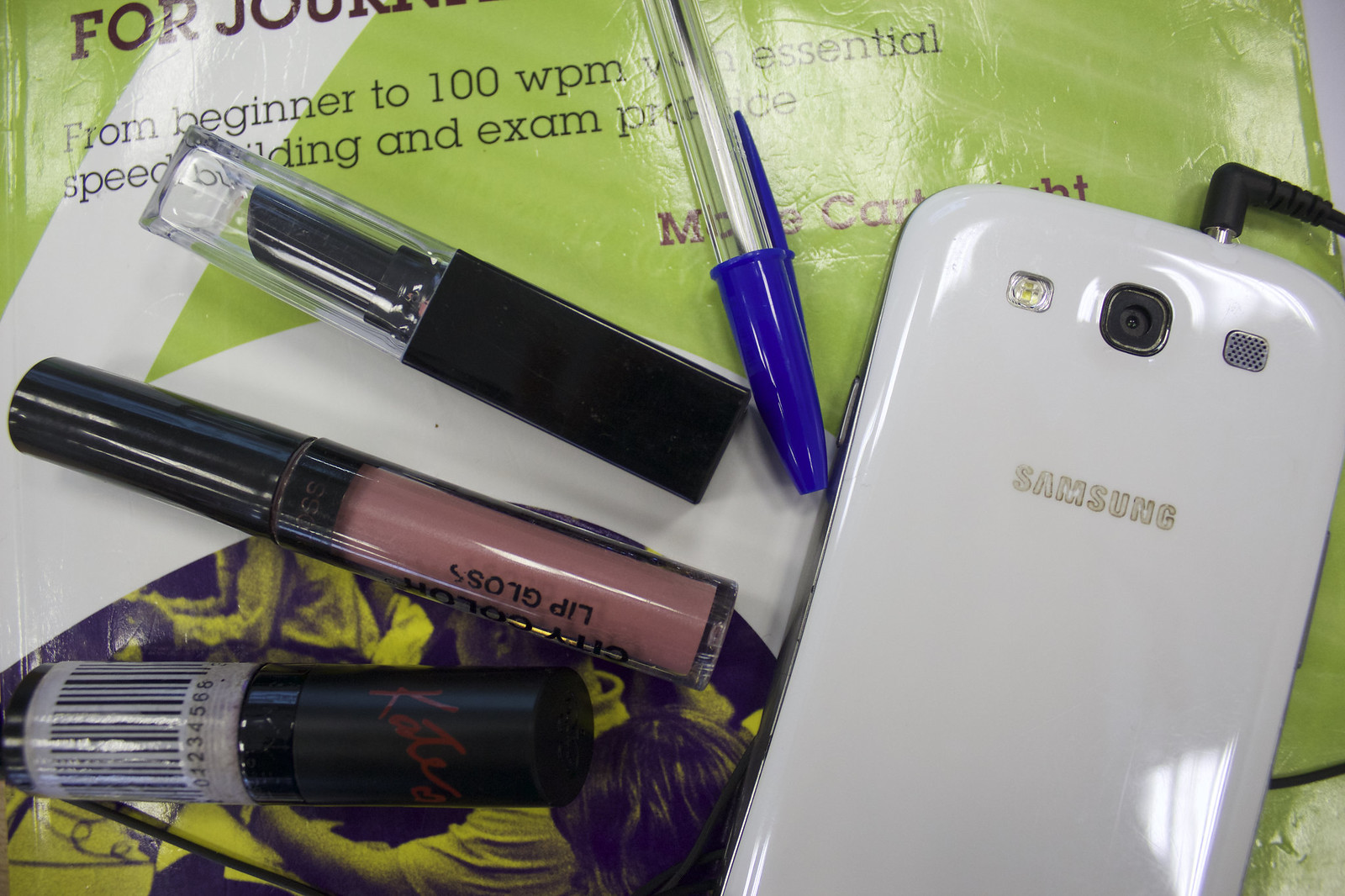The image depicts a neatly arranged collection of items commonly found in a woman's purse, all placed atop a green educational textbook. The visible text on the book reads, "For...from beginner to 100 WPM, essential speed building and exam practice." A white Samsung phone, oriented upside down with a headphone jack plugged in, serves as the centerpiece. Next to the phone lies a blue-capped pen. Surrounding these are three cosmetic items: lip gloss, lipstick, and what appears to be an eyeliner pencil, adding a touch of everyday elegance. The lime green book, featuring white stripes and a lower-left corner adorned with a yellow-tinted photograph of people, is complemented by a second book slightly visible beneath it. Altogether, the items create a meticulously detailed snapshot of personal belongings, suggesting both educational and beauty routines.